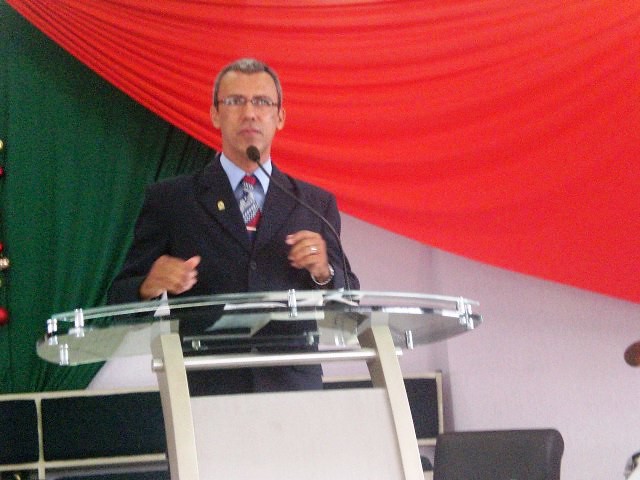This photorealistic image captures a man standing at a podium, likely speaking at an event. The man, who has short, graying black hair and light-colored skin, is dressed in a black suit, a light blue shirt, and a multicolored tie featuring red, blue, white, and black patterns. He also wears black-rimmed glasses and a gold pin on the lapel of his suit jacket.

The podium he stands behind has a silver base with a round glass top and a black microphone. The man holds both hands up near his armpits, gesturing as he speaks. In the background, various drapes in white, red, and olive-green are layered, with the red drape stretching from the top left corner to the middle right side of the image. Near the bottom left-hand side behind him, a black and white shape is visible. The setting appears to be indoors, and the scene is likely captured by a professional photographer.